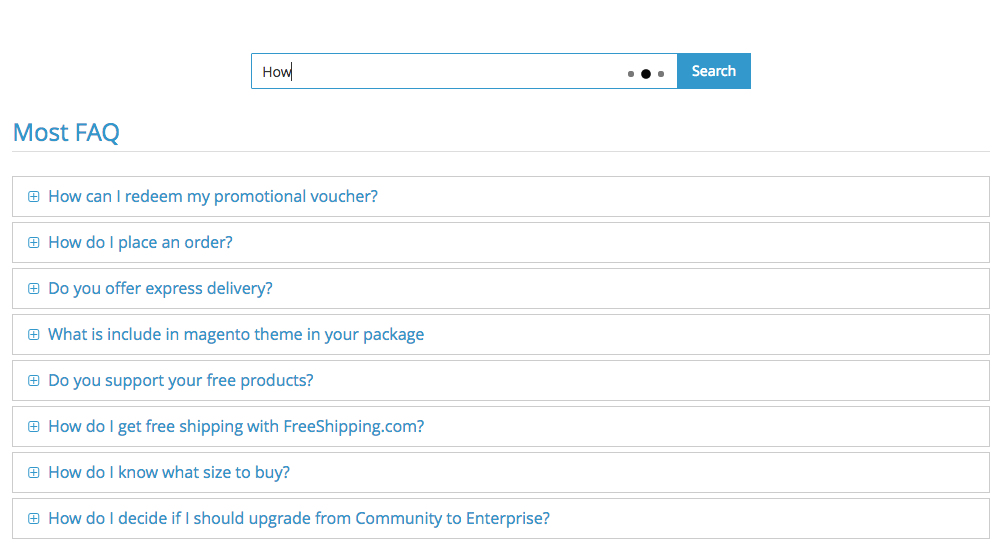Screenshot depicting an interface on a white background. Dominating the top of the image is a search bar with the text "how" followed by a blinking cursor. Adjacent to the search bar are three dots, with the middle dot highlighted in black. Below the search bar is a prominent blue rectangle with the word "Search" displayed in white text.

Beneath this search feature, a list of frequently asked questions (FAQs) is presented. The FAQs include:
1. "How can I redeem my promotional voucher?"
2. "How do I replace or how do I place an order?"
3. "Do you offer express delivery?"
4. "What is included in the Magento theme in your package?"
5. "Do you support your free products?"
6. "How do I get free shipping with freeshipping.com?"
7. "How do I know what size to buy?"
8. "How do I decide if I should upgrade from Community to Enterprise?" (Note: This question appears to be listed twice.)

This clear and structured layout suggests a user-friendly interface designed to enhance the search experience by quickly connecting users with the most relevant information.